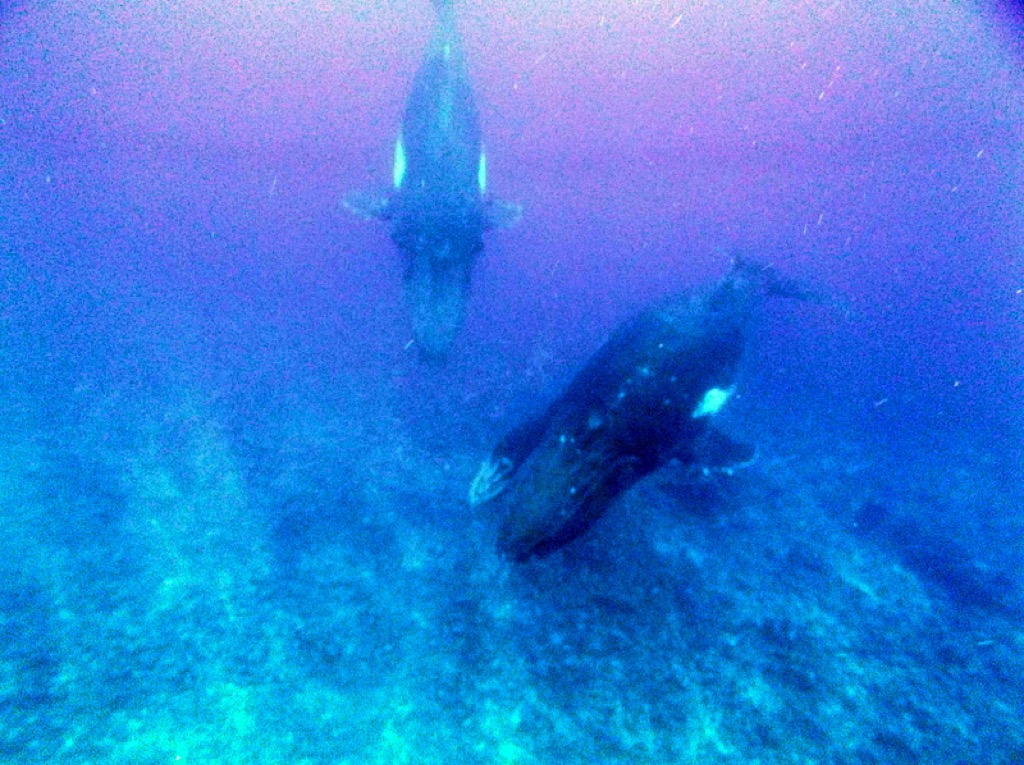This underwater image captures a serene, albeit grainy and slightly out-of-focus, scene with a deep blue backdrop tinged with purplish light from above. At the center of the frame are two whales—potentially a mother and its calf—swimming towards the jagged ocean floor, both facing downward. These whales, likely blue whales or humpback whales, have elongated, rounded noses and long bodies adorned with distinctive white spots on their sides. Their fins are extended, and their tail movements are visible, adding to the dynamic feel of their descent. Though the scene is somewhat dark and blurry, the image effectively conveys the sense of depth and tranquility of the underwater world.